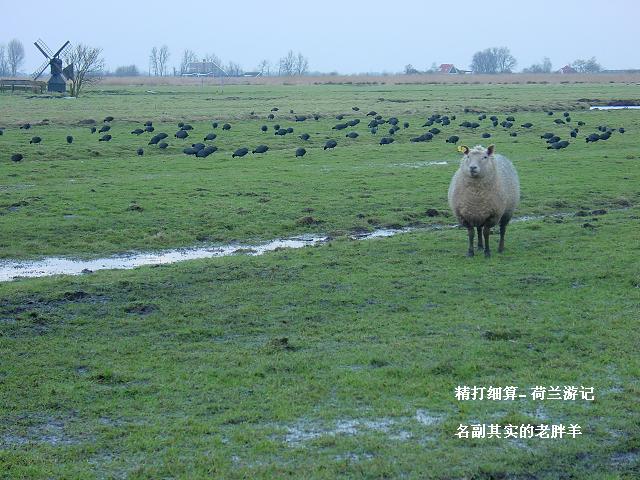The photograph captures a white sheep standing in the foreground of a partially flooded green field, its black legs contrasting with its woolly body. The sheep, facing the camera, sports a yellow tag in its right ear and appears quite calm. Scattered across the field behind the sheep are approximately 50 black birds, possibly turkeys, adding depth to the scene. Further back, a small four-post black windmill stands to the left, with outlines of houses and trees faintly visible in the hazy, light blue-gray sky. Additionally, visible in the bottom right corner, there is white Chinese text.